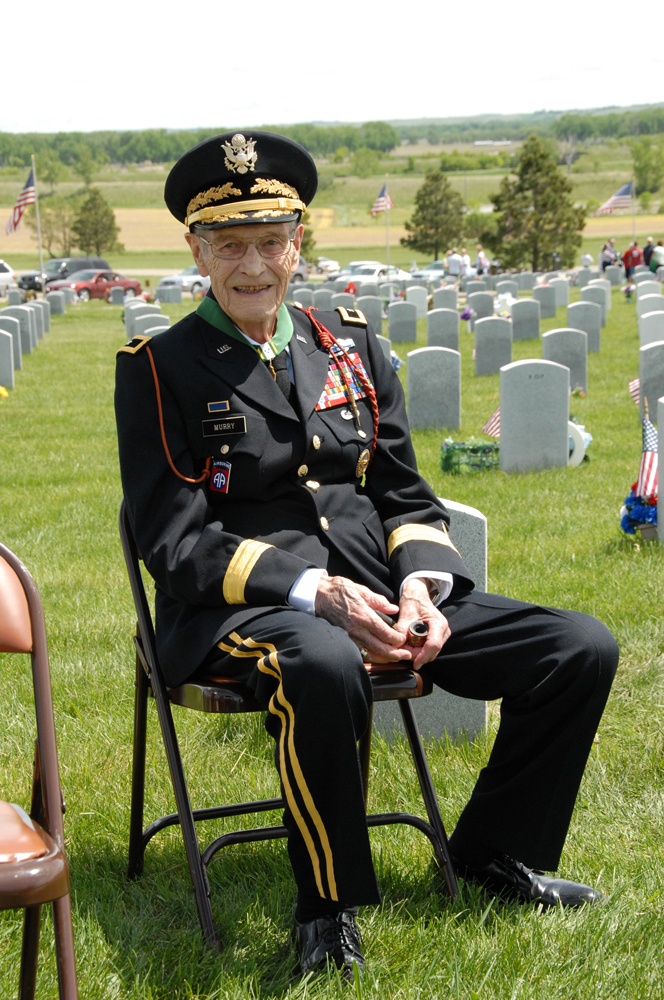In this vertical rectangular image, an elderly white man sits solemnly in a dark brown, almost black folding chair on a grassy expanse of a military cemetery. The scene is set in the daytime with lush green grass underfoot, trees in the distance, and several cars parked in the background. The cemetery is filled with rows of identical white tombstones, each with a domed top and some adorned with small American flags. Larger American flags on poles are also visible among the trees.

The man, who appears to be in his 80s or 90s, dons a striking black military uniform adorned with numerous medals and patches on his chest, and gold stripes running down the sides of his pants and sleeves. His uniform includes a name badge that reads “Murray” on his left chest and multiple badges on his right. He wears a black military hat decorated with a gold eagle emblem and a gold filigree strip above the brim. His face and hands show the wear of age with many lines, and he sports glasses that frame his eyes. Cradled in his hands is a pipe, and he smiles gently, possibly reflecting on his long years of service.